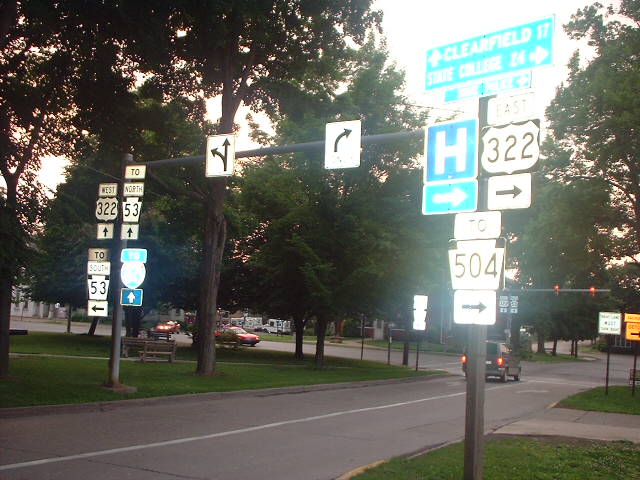This detailed cityscape photo captures a bustling city center with an abundance of greenery and mature, leafy trees lining a wide boulevard. The perspective appears to be from a pedestrian’s viewpoint, perhaps standing at a crosswalk. The photograph features multiple street signs supported by two vertical poles, connected by a horizontal banner above the intersection.

Key details include:

- **Directional Signs**: Two lanes with clearly marked instructions; the right lane indicates 'right turn only,' while the left lane allows for either going straight or making a left turn.
 
- **Highway Indicators**: Prominent signs for highways and routes. Highway 322 West and Route 53 North both continue straight ahead, while Route 53 South requires a left turn. 
 
- **Local Street Names**: Green-background signs specify 'Clearfield Street' straight ahead and 'College Road' to the right. An adjacent sign includes a hospital icon with an arrow pointing left.
  
- **Additional Route Information**: Signs indicating Highway 322 to the right and Highway 504 also to the right, along with markers for a detour and other lower street indicators visible in the background.

The image also captures urban activity with two cars: a minivan halted at a red light at the central intersection, and a smaller red car on the cross street. Benches and a well-maintained park area with lush grass occupy the surroundings, further emphasizing the pedestrian-friendly environment.